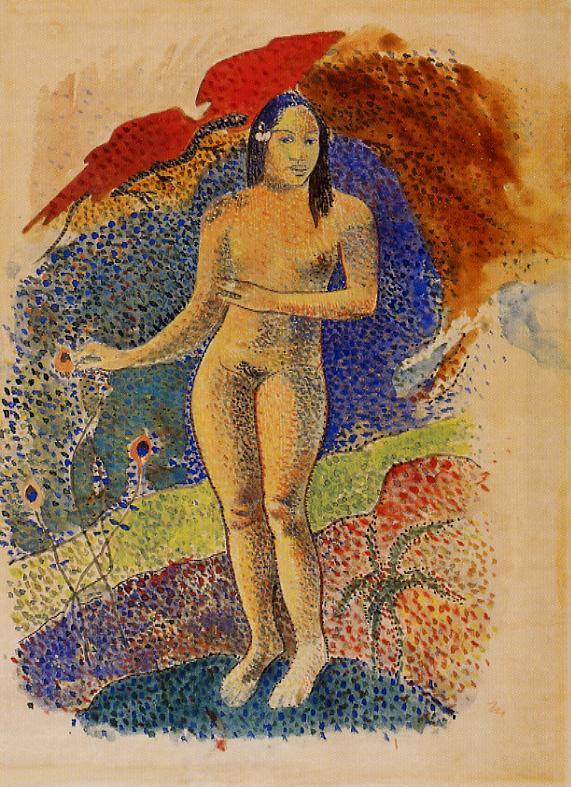This painting, reminiscent of Gauguin's style, features a centrally positioned, nude aboriginal woman rendered in muted, darker tones. She has straight, shoulder-length dark hair, with one arm across her chest and the other extended as if pinching a flower in her hair. Her dark eyes and eyebrows are prominent against the subtle shading of her body. The background is a vibrant mix of swirling blues, browns, and reds, with a profusion of impressionistic and pointillist elements, including flowers, likely peacock feathers, and starfish. A black gecko-like figure is subtly integrated into the composition, climbing a rock-like structure in the top left. The overall scene is enhanced by a harmonious blend of blues, greens, reds, and chestnut tones, with dots used to create shadows and depth, adding to the painting's intriguing and somewhat abstract dimension.